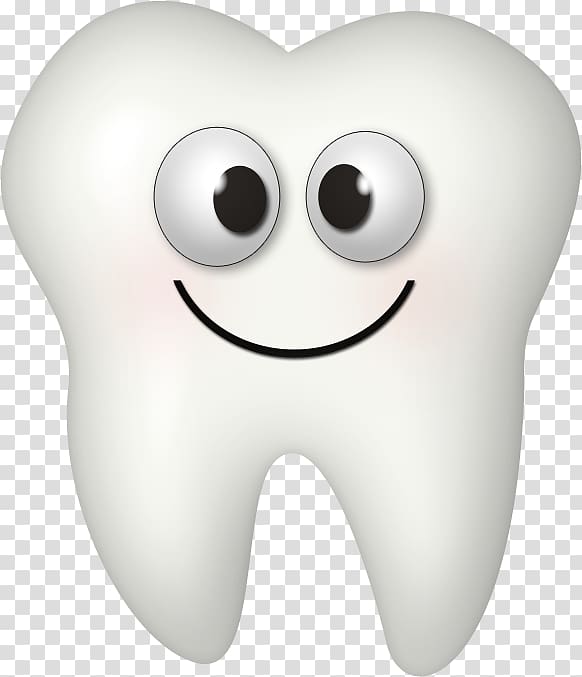This image is a cartoon graphic of a tooth, presented in a rectangular frame where the length of the left and right sides is twice that of the top and bottom sides. The background features a gray and white checker pattern, a common indicator for transparency in image editing. The tooth itself has a cartoon-like design, resembling a molar, with two inward-curving pointed ends at the bottom and two semi-round ends at the top, similar to the top of a heart.

The tooth is predominantly white with dark gray edges. Its charming, humanoid characteristics include a large, downward-curved black smile and two large oval eyes. Each eye has a black pupil positioned inward, giving the tooth a cross-eyed, humorous expression. This playful aesthetic is further enhanced by subtle rosy cheeks, making the design suitable for a setting like a child's dental office.